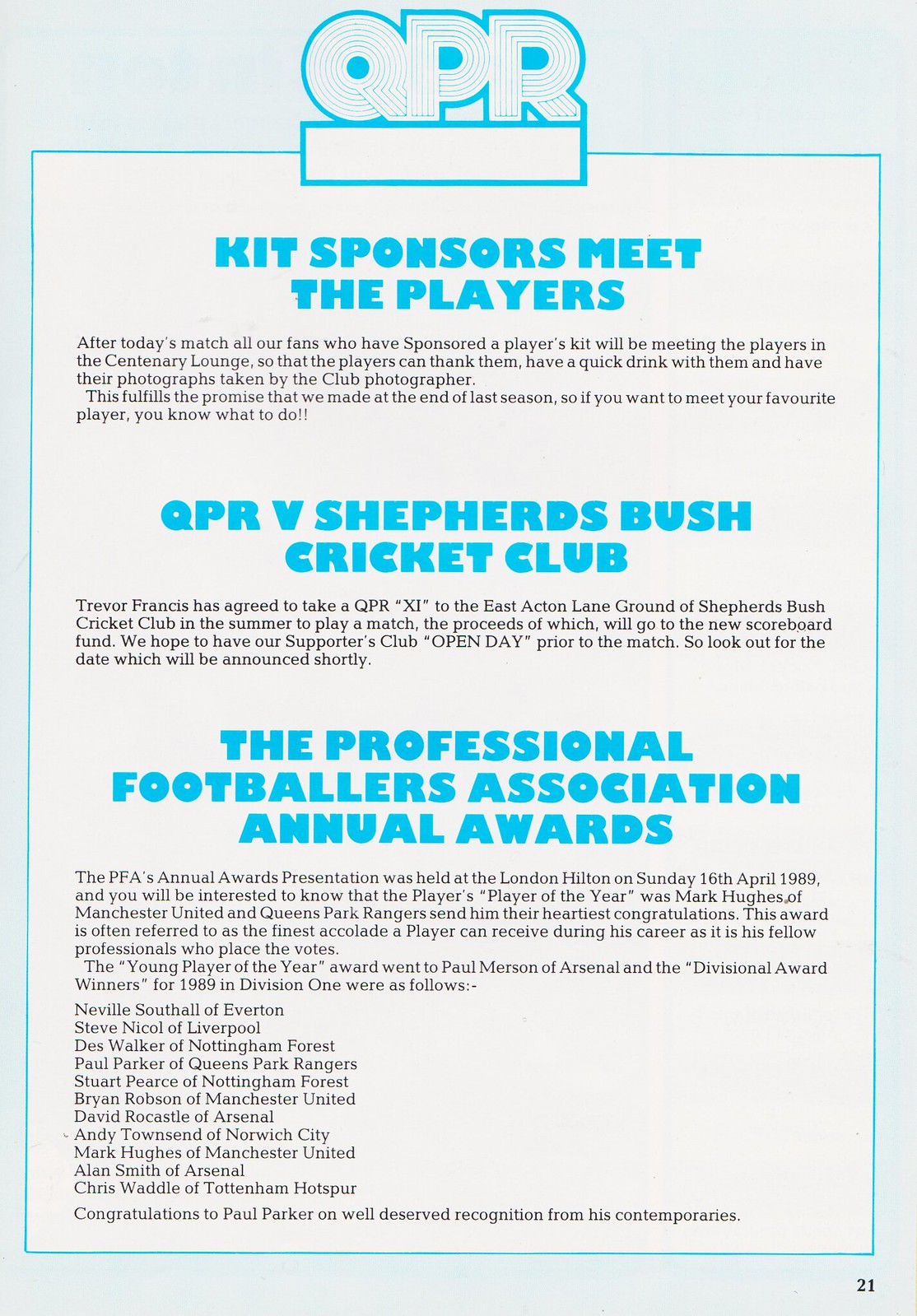The image is a page from a magazine with the number "21" in black font located in the bottom right corner. The page features a light blue background and a white rectangular box in the middle, which is outlined in light blue. At the top of this box are the letters "QPR" in dark blue font, surrounded by concentric circles. The content within the box includes multiple sections each marked by a bold, dark blue headline, and followed by paragraphs of black text.

The first section, titled "KID SPONSORS MEET THE PLAYERS," describes an event taking place after today's match where fans who have sponsored a player will meet the players in the Centenary Lounge. The event promises opportunities for fans to thank the players, have a quick drink with them, and take photographs with the club photographer. This initiative fulfills a promise made at the end of the last season.

The second section headline reads "QPR THE SHEPHERDS BUSH CRICKET CLUB." It details an upcoming summer match where Trevor Francis will lead the QPR Eleven to play against Shepherds Bush Cricket Club at East Acton Lane ground. The match proceeds will go towards a new scoreboard fund and there is a planned supporters' club open day prior to the match, with the date to be announced soon.

The final section is titled "THE PROFESSIONAL FOOTBALLERS ASSOCIATION ANNUAL AWARDS." The paragraph underneath informs readers about the PFA's annual awards presentation held at the London Hilton on Sunday, April 16, 1989. Mark Hughes of Manchester United was named the Players' Player of the Year, receiving high praise as this award is voted on by fellow professionals. The Young Player of the Year award went to Paul Merson of Arsenal. The section concludes with a list of divisional award winners from Division One in 1989, including notable names such as Neville Southall, Steve Nicol, Des Walker, Paul Parker, Stuart Pearce, Brian Robson, David Rocastle, Andy Townsend, Alan Smith, Chris Waddle, and recognizes Paul Parker's well-deserved accolades.